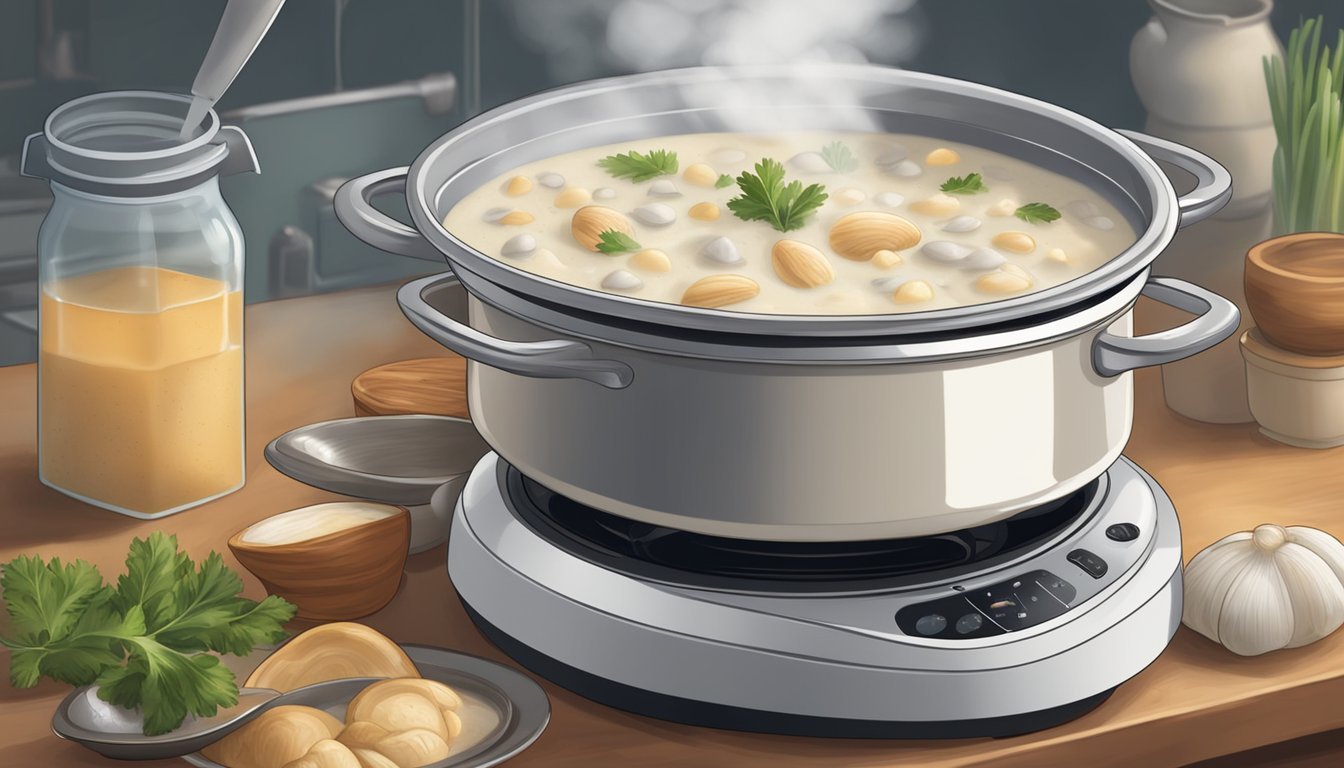This is a horizontally aligned, digitally generated artwork depicting a crockpot on a brown wooden counter. The silver crockpot consists of a bottom and top portion, each with silver handles. The crockpot contains a light yellow, creamy broth with floating green leaves, brown oval shapes resembling nuts, and white chunks. Steam can be seen rising from the pot. To the left, there is an open jar with a utensil inside, filled halfway with a light brown liquid. Nearby, there are more green leaves, additional brown pieces, a sliced coconut, and what seems to be a clove of garlic. On the right side, there's an onion, various wooden bowls, and what appears to be celeriac. The scene captures a detailed and vibrant kitchen environment.